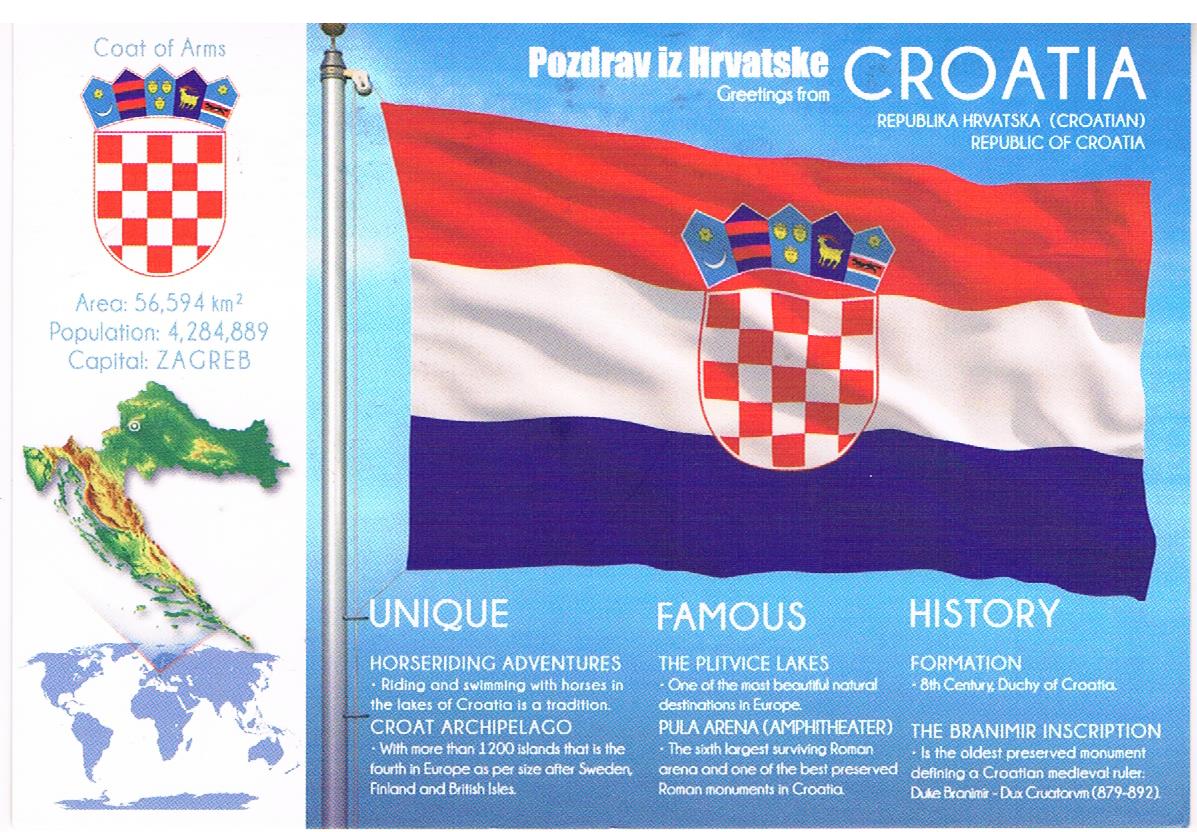This image appears to be a detailed postcard or souvenir card from Croatia. On the right side, it prominently features the Croatian flag, which has three horizontal stripes: red on the top, white in the middle, and blue on the bottom. In the center of the flag is a checkered shield, the Croatian coat of arms, topped with five smaller shields depicting historical regions. The flag is held by a silver pole indicating it is flying to the right. Above the flag, white text reads "Pozdrav iz Hrvatske" (Greetings from Croatia), "Republika Hrvatska" (Republic of Croatia). 

On the left side of the image, a white band provides additional information about the Croatian coat of arms, detailing its red and white checkered pattern and historical significance. Below this, the card features a small map highlighting Croatia's position within Europe and the world.

Underneath the flag, the card is divided into three columns. The first column, labeled "Unique," highlights activities such as horse riding and swimming with horses in Croatia's lakes, emphasizing it as a traditional practice. The second column, "Famous," likely provides two notable facts about the country's fame. The third column, "History," shares historical insights, including Croatia being home to more than 1,200 islands, making it the fourth largest archipelago in Europe, after Sweden, Finland, and the British Isles.